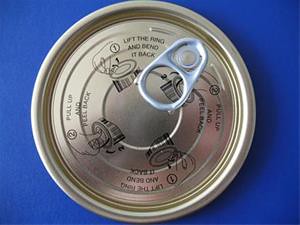On a blue background, a small, circular pull-tab can resembling a tuna can is prominently displayed. The can itself is a light yellow-gold color, providing a striking contrast to the blue backdrop. Positioned at around the 2 o'clock mark on the can's surface is a silver pop-tab pull tab. Surrounding the pop tab are printed instructions detailing the opening mechanism. On the left side of the tab, step one instructs to "Lift the ring and bend it upward," and step two follows with "Pull up and peel back." These instructions are stamped in a repeating sequence, making the usage instructions clearly visible and easy to follow.